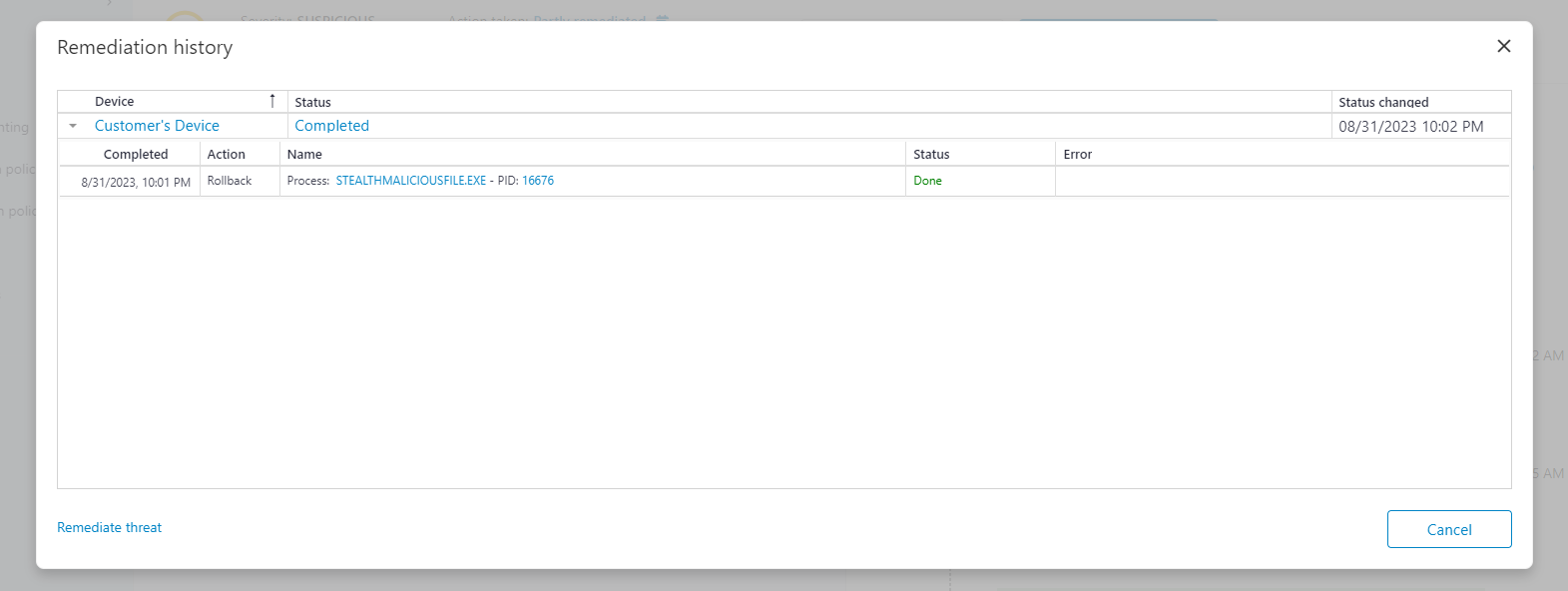The screenshot depicts a pop-up menu with a white rectangular background bordered by grey. At the very top in the upper left corner, the title "Remediation History" is displayed in black font. In the upper right corner, there is a small "X" icon for closing the menu.

Beneath the title, there are several black-outlined rectangles arranged in rows. In the upper left of these rectangles, the word "Device" is displayed next to an upward-pointing arrow. Adjacent to this, a new bar labeled "Status" appears, followed by another labeled "Status Changed."

Below these headings, in blue font, it shows "Customer's Device" next to the status "Completed." The timestamp "08-31-2023 at 10:02 PM" is also listed there.

Further down, there's another set of labels: "Completed," "Action," "Name," "Status," and "Error." Under "Completed," it reads "08-31-2023, 10:01 PM." The action taken is documented as "Rollback," and it involves the process "stealthmaliciousfile.xpc16670."